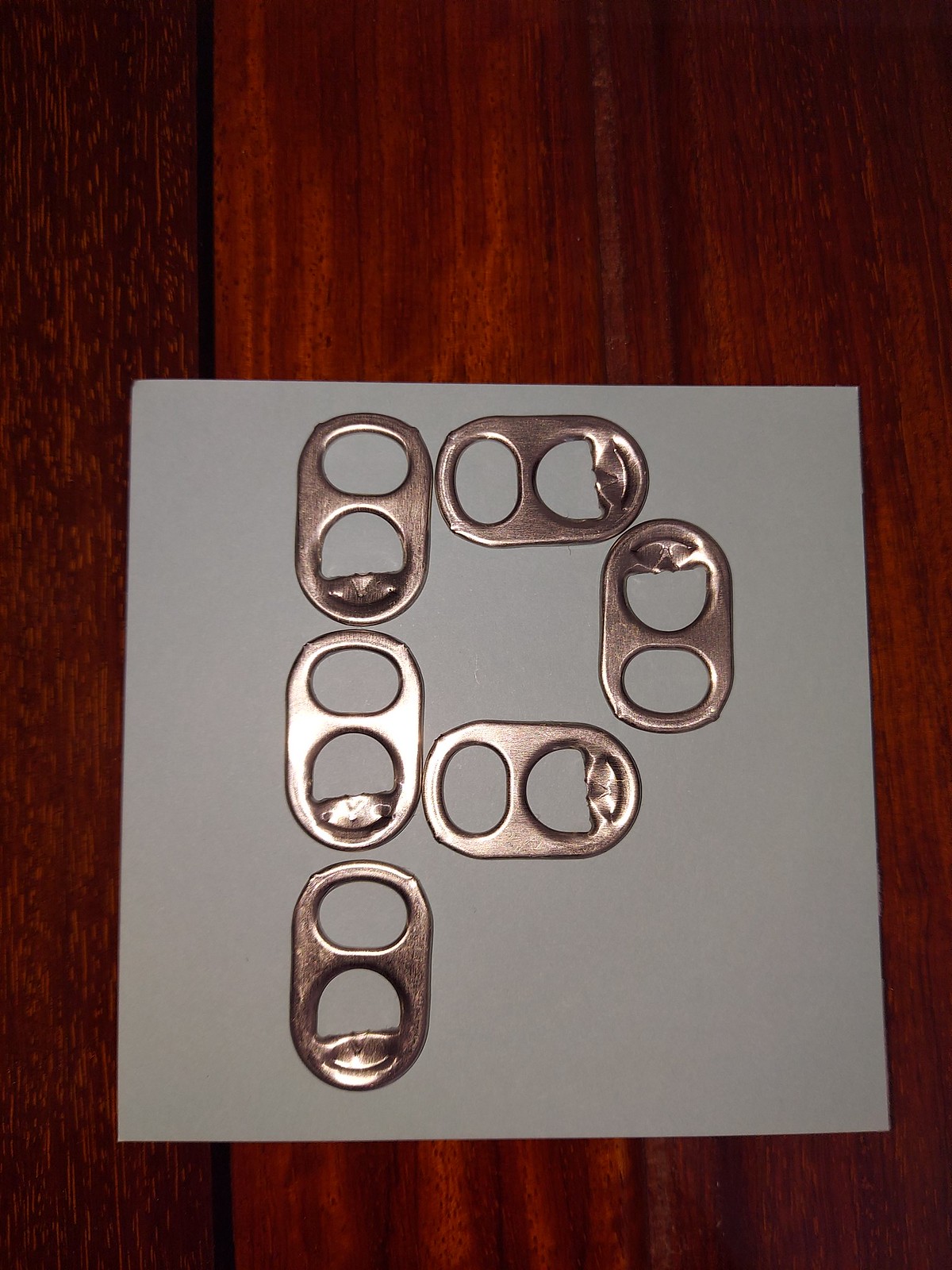This detailed color photograph captures a close-up view of a dark brown polished wooden surface with intricate reddish and chocolate brown streaks, likely a type of red oak. Resting on this elegant wood is a light blue square of construction paper. On top of the paper, six silver aluminum pull tabs are meticulously arranged to form a lowercase "p." The pull tabs, each identical in size and shape with two round cutouts, reflect the overhead lighting, creating a subtle metallic gleam. The scene is shot in portrait mode, with the camera positioned directly above, emphasizing the textures of both the wood grain and the glossy pull tabs.